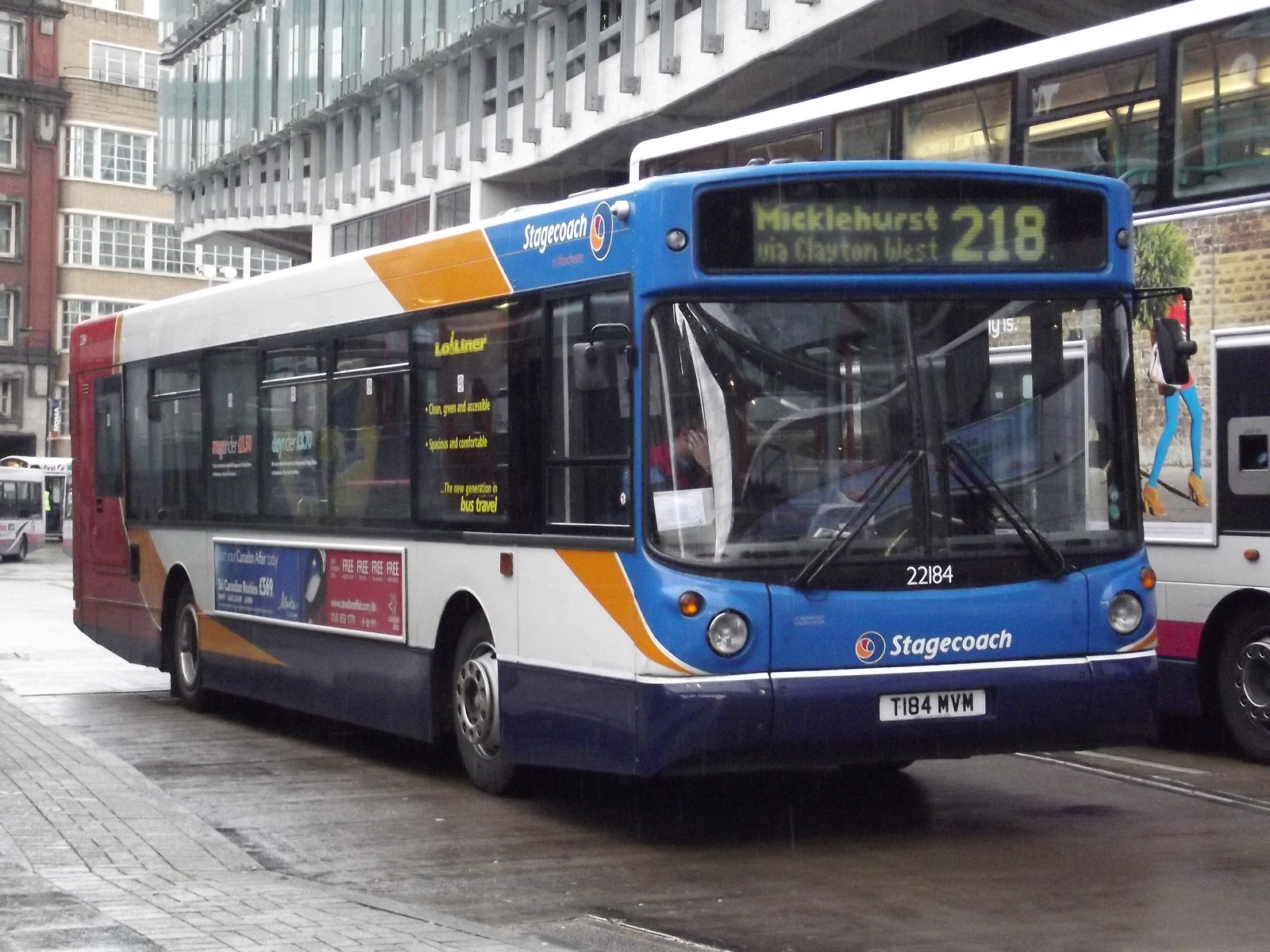This image features a multi-colored transit bus captured from a front-right angle on a small city street during the daytime. The bus prominently displays a blue front panel with the Stagecoach logo at the bottom, transitioning to yellow, white, and red along the sides. It is identified as route number 218, "Micklinhurst via Cloran West," and bears the number 22184 and license plate T184 MVM. The large windshield is reflecting light, and the bus carries advertisements in metal frames on its sides—one blue and one red.

The city street is narrow, lined with multi-story buildings closely surrounding the bus; a green building sits to one side and a beige building behind it. The sidewalk is visible. The wet road surface suggests recent rain, as indicated by the reflective sheen. A mostly obscured double-decker bus is positioned to the right of the main bus. Overall, the scene captures a vibrant street environment centered around this colorful public transit vehicle in a European urban setting.